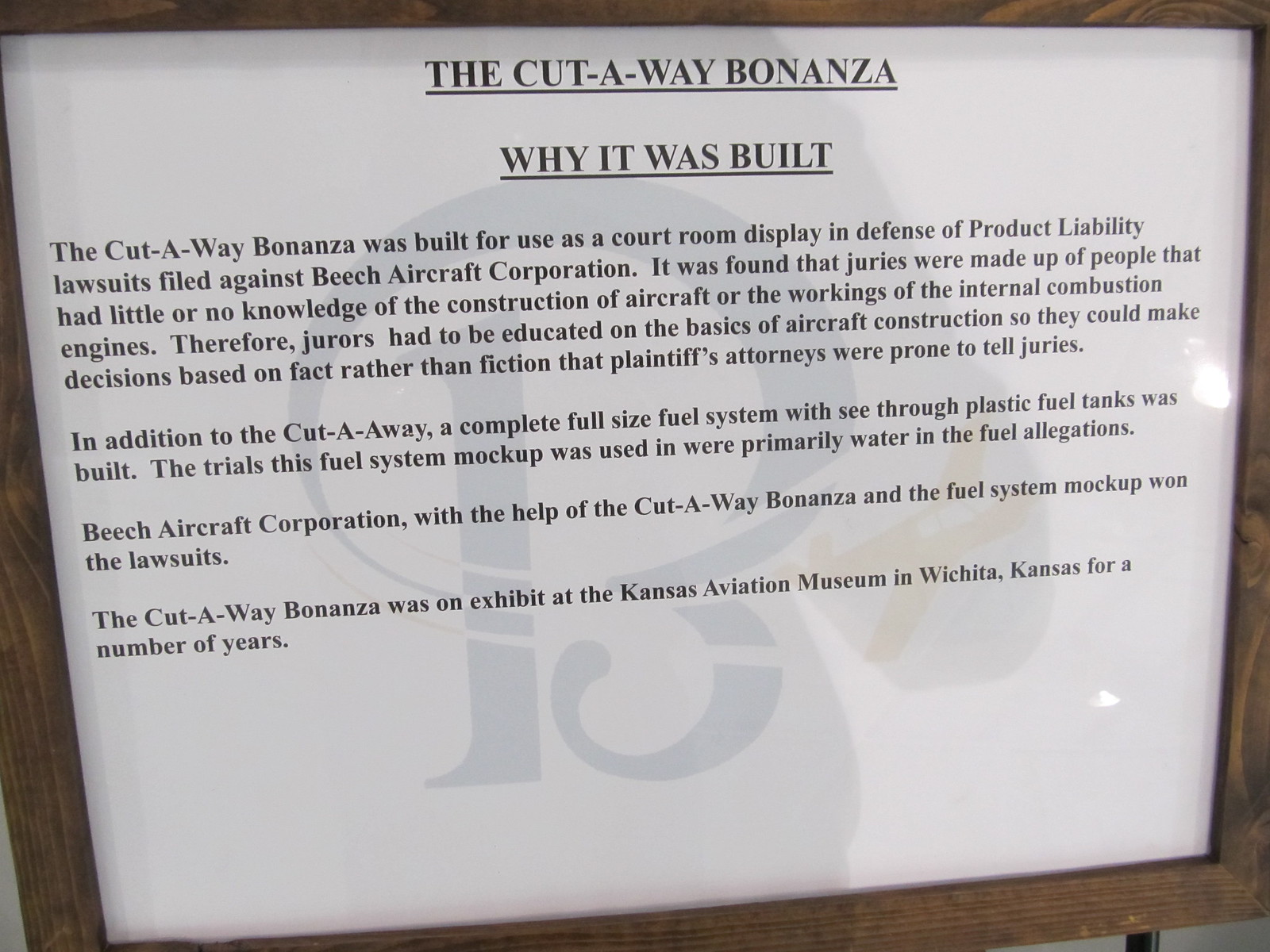The image showcases a close-up of a museum placard with a predominantly white background, encased in a dark brown wooden frame with visible grain. The placard features a light blue watermark of a manufacturer's logo with a light yellow airplane graphic in the background. The title, written in black text, reads "The Cutaway Bonanza" followed by the subheading "Why it was built." The document explains that the Cutaway Bonanza was created as a courtroom display for Beach Aircraft Corporation to defend against product liability lawsuits. It highlights the need to educate juries, who often had little to no understanding of aircraft construction, about the basics to make informed decisions. The placard mentions that a full-size fuel system mock-up with see-through plastic tanks was also built and used primarily in trials involving fuel allegations. Both the Cutaway Bonanza and the fuel system mock-up played a crucial role in winning these lawsuits. The Cutaway Bonanza was on exhibit at the Kansas Aviation Museum in Wichita, Kansas, for many years. The sign has a shiny, reflective coating, evidenced by the reflection of a light bulb on its right side and another bright spot further down. Additionally, the shadow of a man, cast by lights coming from behind the photographer, is visible on the placard.